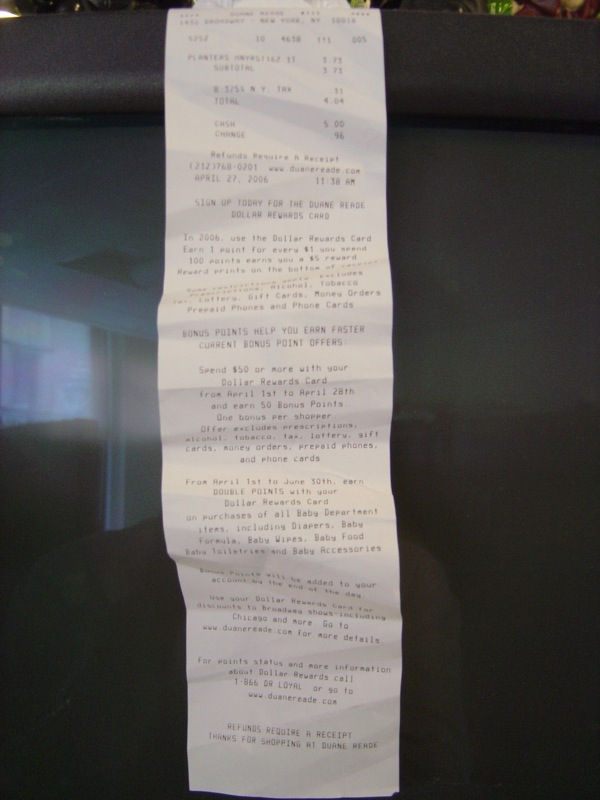The photograph captures an extremely long white receipt with black print, draped over the side of a gray couch. The image quality is poor, making the text difficult to read. Despite this, some details are discernible. The receipt features a charge with a stated total of $4.04, a cash payment of $5.00, and change given as $0.96. There are numerous mentions of rewards and bonus points, including a "Dollar Rewards Program." Phrases like "planters," likely referencing Planters peanuts, and "sign up today" are visible. The receipt indicates a purchase date of April 27, 2006, at 11:38 AM, and includes instructions and benefits related to the rewards card, such as earning points for every dollar spent and additional bonuses for specific purchases. The receipt also emphasizes the store’s refund policy, noting that refunds require the original receipt. Despite the ambiguity caused by the image quality, it's evident that the receipt is from DuMoine REIT.